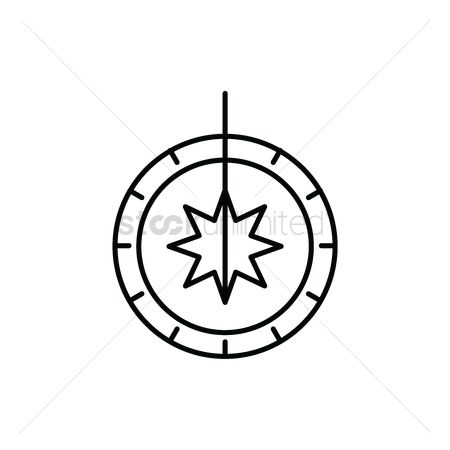The image features a distinctive logo set against a white background. At its core, there are two concentric black circles, with the smaller circle nested inside the larger one. The outer circle is encircled by tiny black lines placed at regular intervals, resembling the markers on a clock face. Inside the smaller circle, an eight-pointed black star emerges, spanning from the bottom to the top of the circle, perfectly aligned with the 12 o'clock position. A prominent vertical line bisects this star, stretching from the 6 o'clock position to the 12 o'clock position, further emphasizing the clock-like structure.

Additionally, four thin gray lines radiate diagonally in an X shape, intersecting the star and extending outward past the circles. The word "limited" is subtly inscribed in gray letters at the top of the image. An intricate detail includes an S-like shape and a T-like line within the circle's arch, contributing to the logo's complexity. Although there is no explicit business name, the image combines these elements to create an intricate and striking logo design.